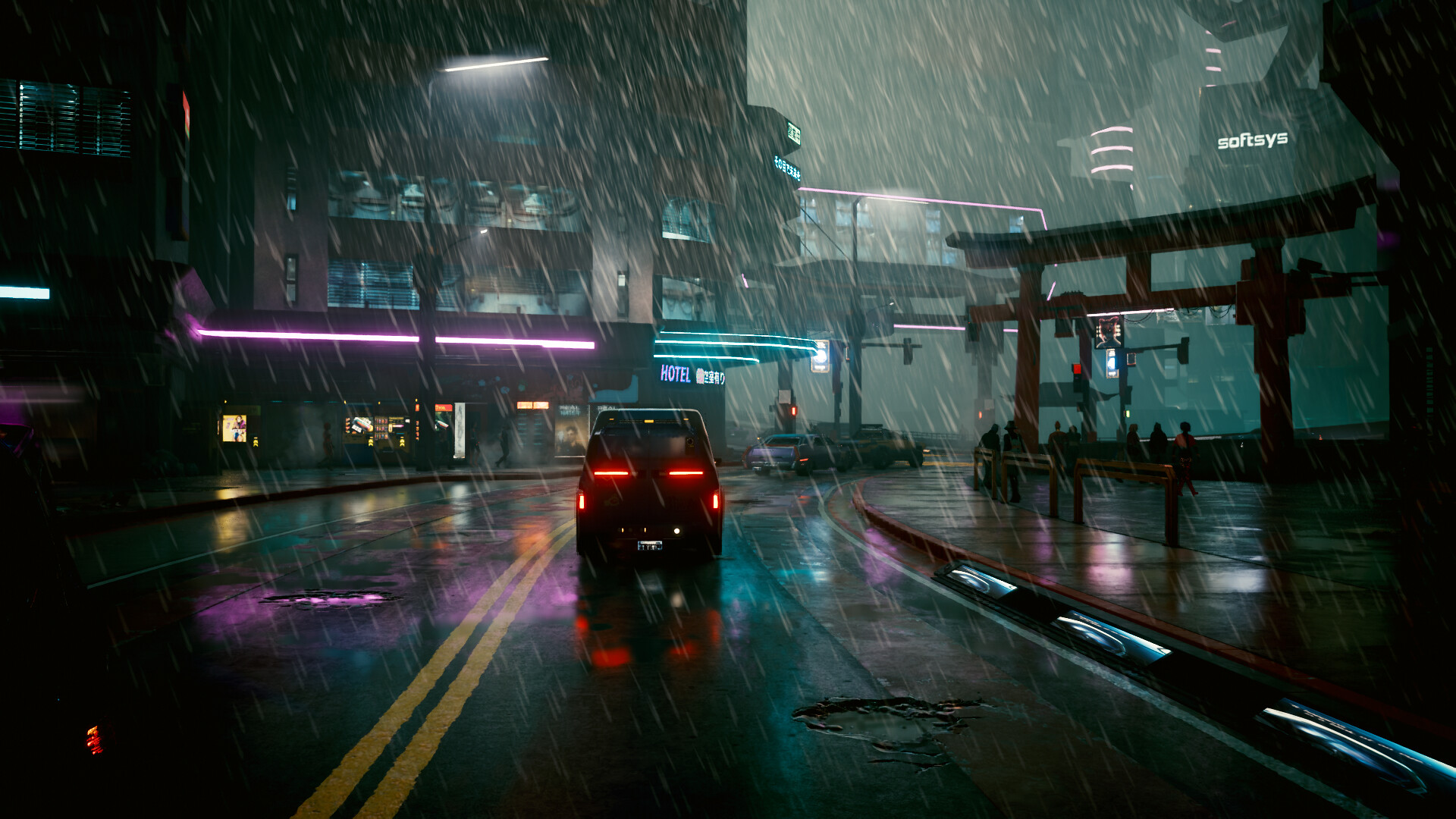A car drives down a dimly lit street in a city at night, as captured from behind the vehicle. The street, divided by a yellow center line, features two lanes and appears to be a backstreet in an urban area. The scene is shrouded in the atmospheric glow of streetlights reflecting off wet pavement, indicating that it is raining. On the left side of the image, a gray building with LED lighting at its base near the awning adds a subtle, modern touch to the setting. To the right, a sidewalk is visible, flanked by buildings in the background that fade into the rainy night, contributing to the melancholic yet serene ambiance of the scene.